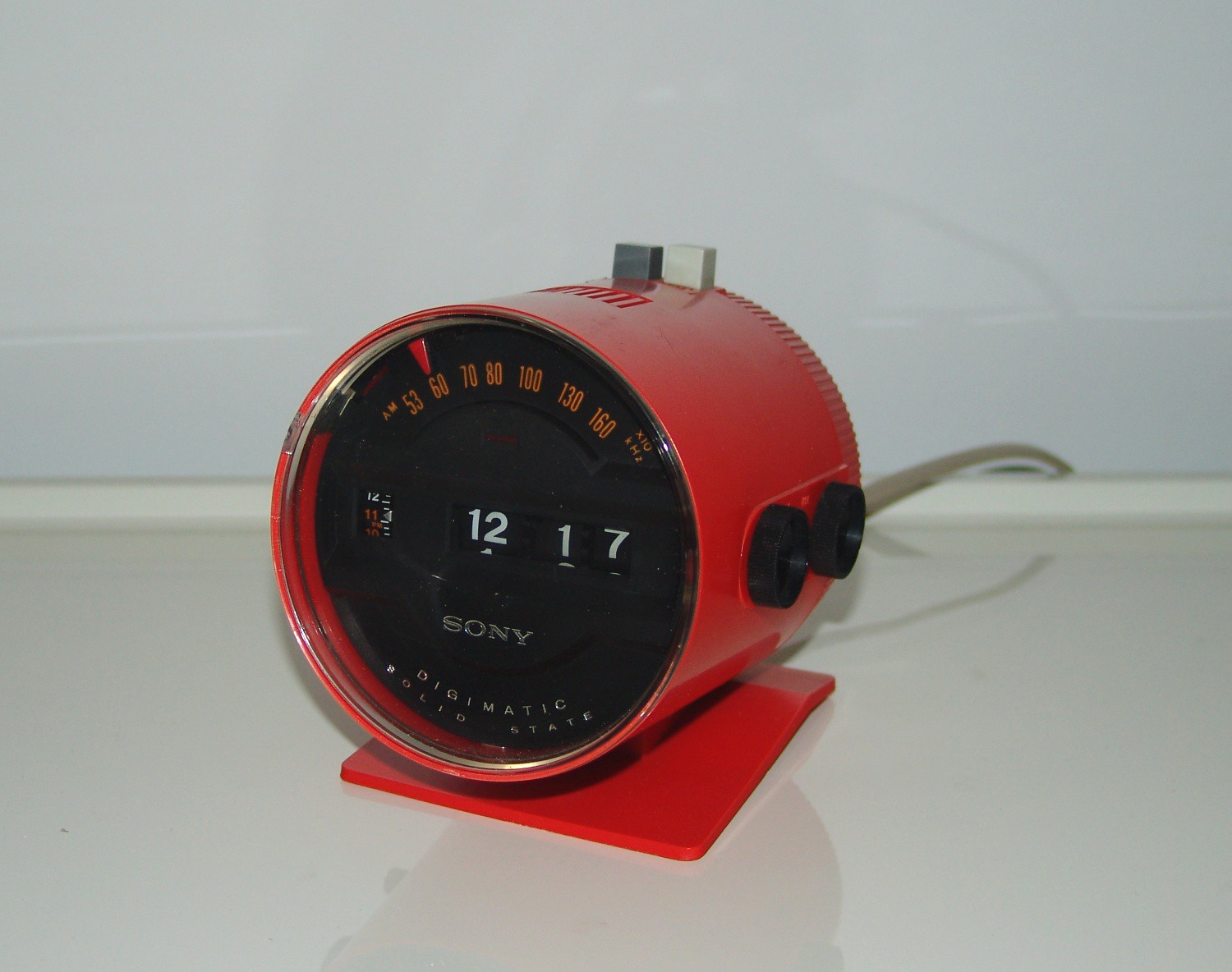The image features a vintage, red Sony Digimatic Solid State clock radio, prominently displayed on a pristine white laminate countertop. The backdrop consists of a plain white wall, providing a stark contrast that highlights the vibrant color of the clock radio. This classic piece of technology, cylindrical in shape, showcases a timeless design.

At the front of the clock, the time reads '12:17' in bold, old flip style numbers, adding a touch of nostalgia. Just above the time display, there is a dial marked with AM frequencies ranging from 53 to 160, indicating the radio functionality. The right side of the device houses two black dials, presumably for setting the clock and tuning the radio.

A distinctive silver handle extends across the top rear of the cylinder, suggesting portability, while an electric cord protrudes from the back, emphasizing its electronic nature. The clock radio rests firmly on the smooth countertop, its metallic sheen and well-preserved condition evoking a sense of timeless elegance.